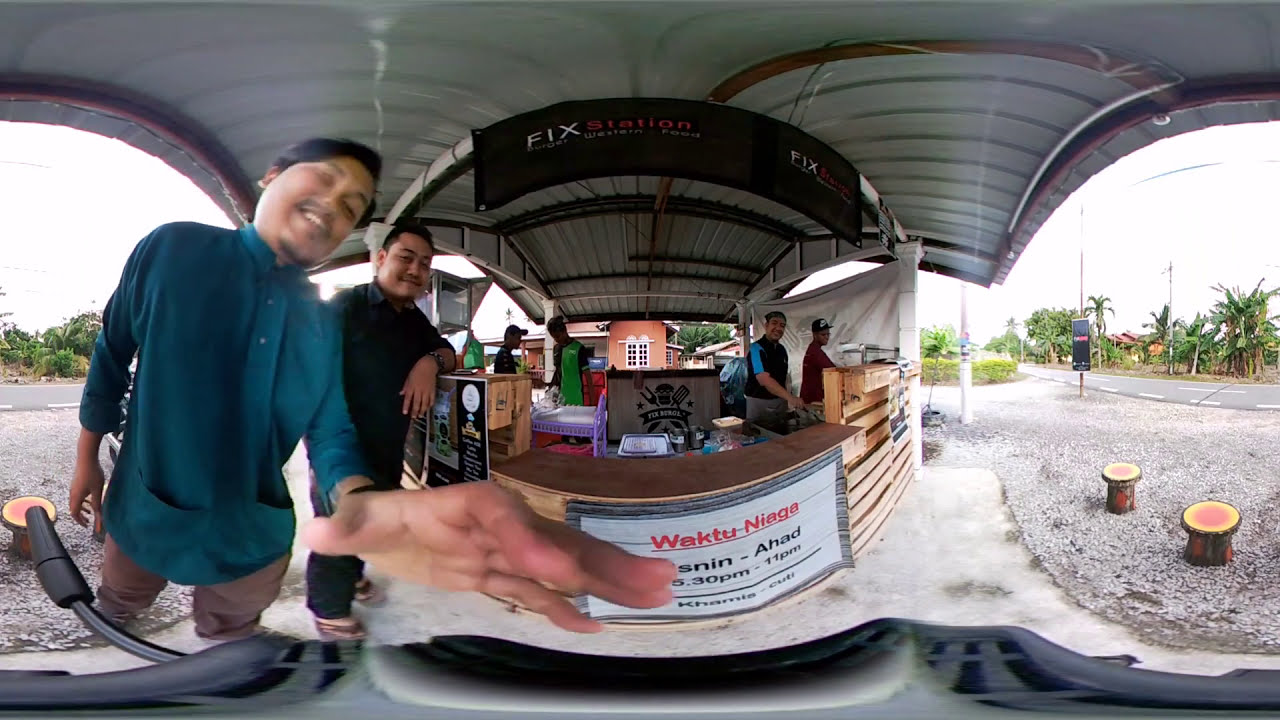The image depicts an outdoor roadside food stall named "Fix Station," with a black sign above reading "Burger Western Food." The stall is constructed from wooden pallets and covered by a metal roof. In the foreground, a man in a blue button-up long-sleeve shirt and tan pants stands with his hand reaching towards the camera, smiling. Behind him, another man dressed in all black leans against the wooden counter. Three more men are visible inside the stall, busy at work.

In front of the stall, there are log-like wooden stools with round red and yellow seats, inviting customers to sit and enjoy their food. A white, black, and red banner hanging in front of the stall displays the operational hours "Waktu Niaga: 6:30 p.m. to 11 p.m." In the distance, you can see a gravel parking lot, a road with power lines, and a row of palm trees, suggesting a tropical location, possibly the Philippines. The entire setting embodies a casual and welcoming roadside dining experience.